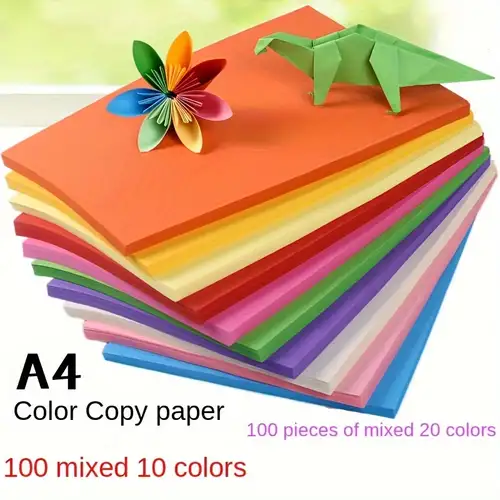The photograph showcases an assortment of colored A4 copy paper arranged in ten small, fanned-out stacks, each featuring a different vibrant color. From top to bottom, the visible colors are orange, yellow, light yellow, red, pink, green, purple, white, light pink, and light blue. Positioned atop this colorful array are two intricate origami figures: a green dinosaur to the right and a multicolored flower composed of various colored paper petals on the left. The image is slightly low resolution but clearly intended as a product photo. Text at the bottom of the image includes "A4 color copy paper" in black, "100 pieces of mixed 20 colors" in purple, and "100 mixed 10 colors" in red. This photo effectively highlights the diversity of color options and the creative potential of the paper.